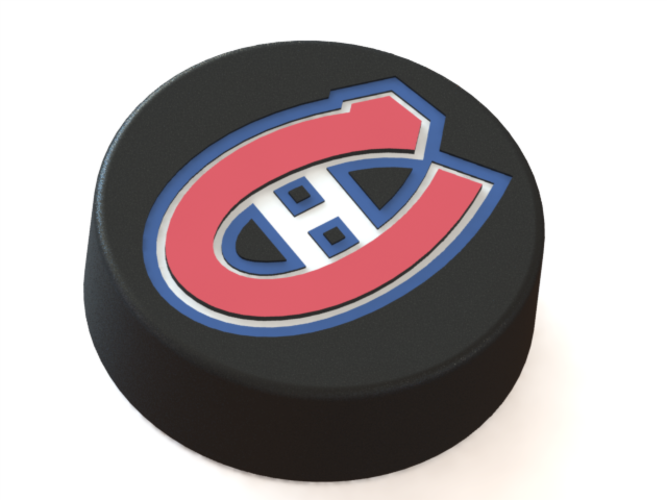The image showcases a detailed digital rendering of a glossy, black, three-dimensional hockey puck with the Chicago Blackhawks logo prominently displayed on its surface. The puck is set against a pure white background, viewed slightly from above and to the side, casting a faint shadow on the bottom right.

On the top and center of the puck, there is a large, bold red letter "C" outlined by successive white and blue borders. Inside the "C" is a white letter "H," which is further outlined in blue, accentuated by small blue and black dots on the upper and lower arms of the "H." The "C" is oriented with its opening facing the top right and its loop toward the bottom left. The detailed layering of colors and outlines within the logo adds a striking contrast against the black surface of the puck, making it a discernible emblem likely representing the Chicago Blackhawks.